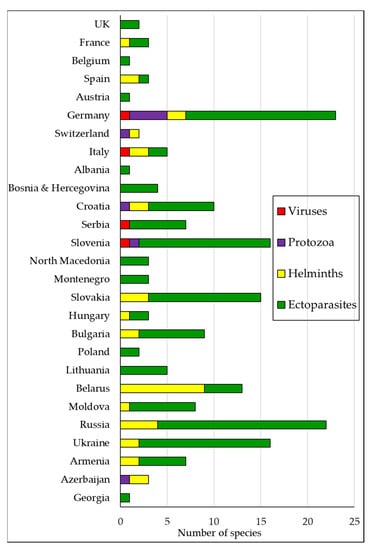The image displays a detailed horizontal bar chart illustrating the distribution of species across various countries. The left-hand side features an extensive list of country names, including the UK, France, Belgium, Spain, Austria, Germany, among others, totaling approximately two dozen. Each bar, extending horizontally to the right, is segmented into multiple colors—green, yellow, red, and purple—each representing a different type of species. Specifically, green denotes ectoparasites, yellow indicates helminths, red signifies viruses, and purple represents protozoa. This color-coded legend is centrally positioned on the right side of the chart for easy reference. Notably, Germany, Russia, and Ukraine exhibit the longest bars, indicating a higher number of species compared to other countries. Additional countries listed include Switzerland, Italy, Albania, Bosnia and Herzegovina, Croatia, Serbia, Slovenia, North Macedonia, Montenegro, Slovakia, Hungary, Bulgaria, Poland, Lithuania, Belarus, Moldova, Armenia, Azerbaijan, and Georgia.